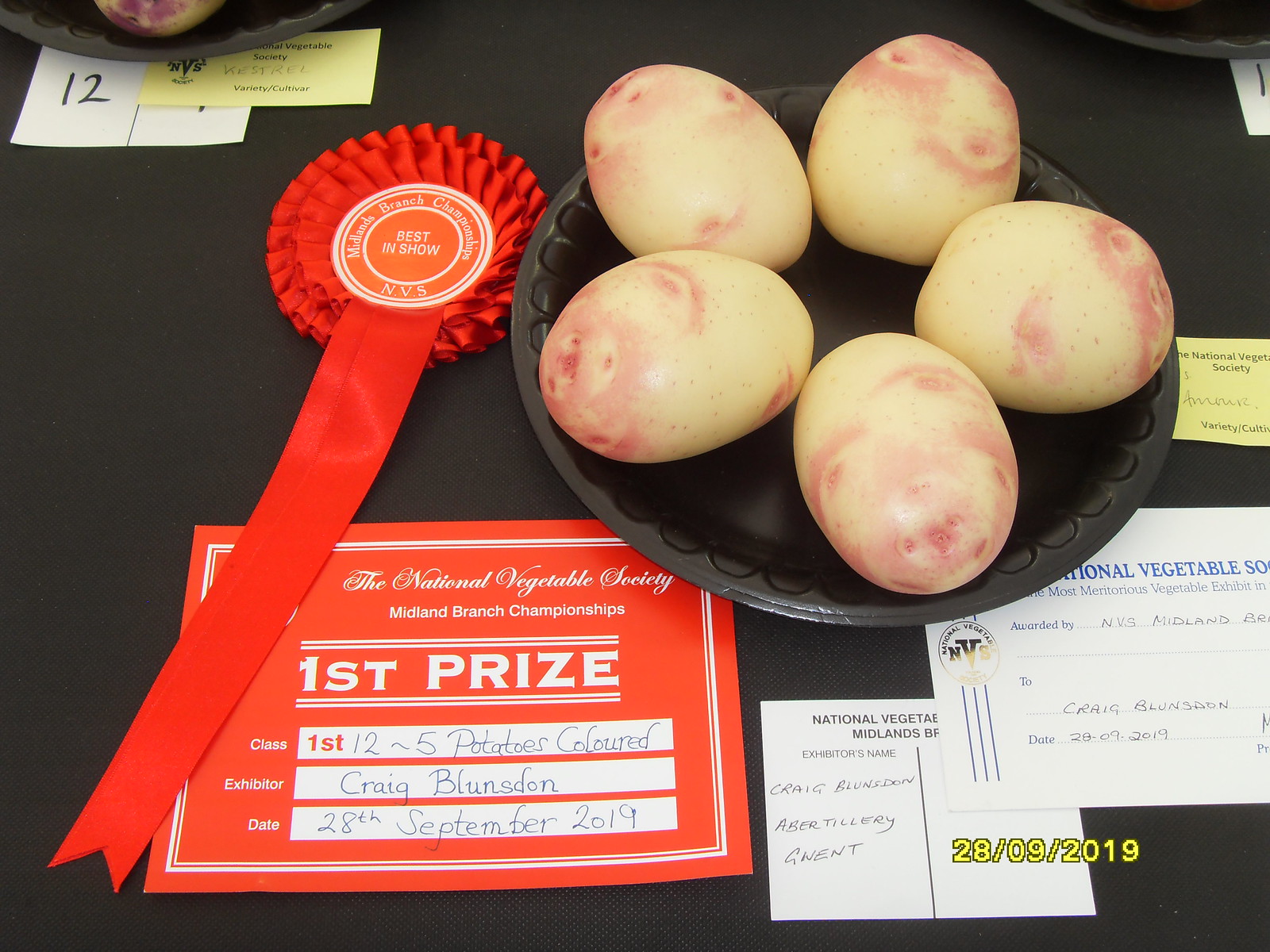The image captures a detailed scene from a food contest, likely a national potato competition. Central to the picture is a black plastic bowl filled with five potato-like objects. Positioned prominently next to the bowl is a red ribbon inscribed with "Best in Show," as well as the letters "NDS." Below this ribbon and the bowl is a certificate or card reading "National Vegetable Society, Midland Branch Championship, First Prize, 12-5 Potatoes, Exhibitor: Craig Blundstown, 28th September 2019," indicating that Craig Blundstown's potatoes won first place. Scattered around these main elements are two or three postcard-sized cards, one of which bears the date "28-09-2019," further confirming the event's details. In the upper left corner, a small yellow business card-sized item is partially visible, adding to the array of presented items. The primary colors in the image include black, red, white, yellow, purple, and blue, all set against what appears to be a black table, suggesting an indoor setting.